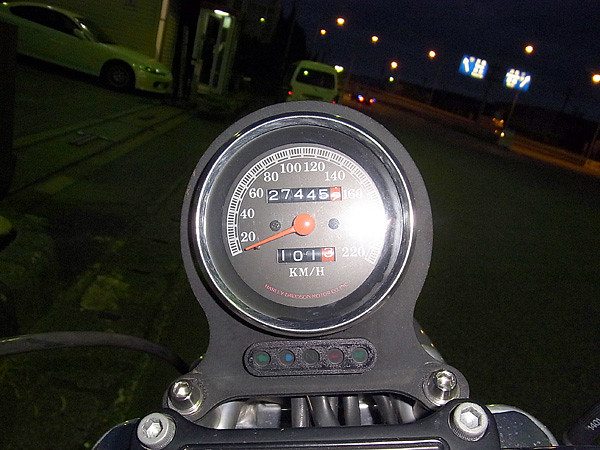This close-up nighttime photograph captures an odometer encased in a black housing with a silver rim and a glass cover. The odometer, bolted to an unseen black structure that could possibly be part of a motorcycle, reveals a reading of 27,445 miles. A red needle rests at zero inside the odometer. 

In the background, the scene extends to a road bordered by a curb. To the left, a parking lot is visible. A white van ahead displays illuminated brake lights, while a white sedan to the left seems poised to exit the parking lot. Further in the distance, street lights dot the landscape, illuminating a highway where cars travel in opposing directions, including a prominent semi-truck.